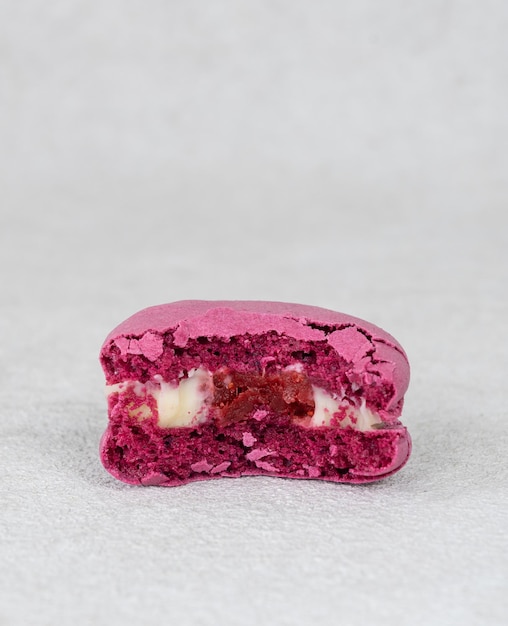A delectable pink macaron, impeccably captured from the side against a pristine white background, gives a glimpse of its tempting interior. The macaron appears to have been broken in half or nibbled on, revealing its soft, textured layers. The top and bottom shells boast a fluffy pink hue, with their edges turning slightly darker, creating a stunning contrast against the paler, almost pastel pink surface. A hint of crumbliness on the edges suggests its delicate nature. Sandwiched between the pink shells is a generous layer of velvety white cream, encasing a lush dark magenta filling, indicative of a fruity flavor likely to tantalize the taste buds. This visually appealing depiction of the macaron makes it a perfect candidate for a menu advertisement, promising a delightful and indulgent treat for dessert enthusiasts.